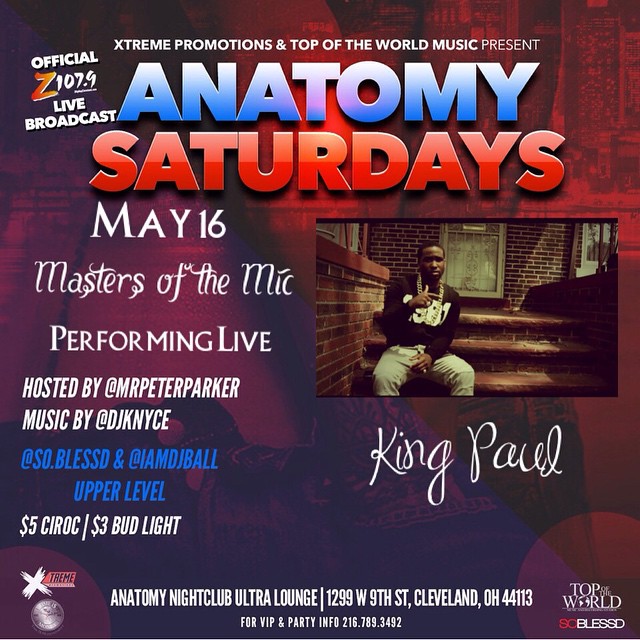This image is a detailed flyer promoting a nightclub event titled "Anatomy Saturdays" presented by Extreme Promotions and Top of the World Music. It features an official Z107.9 live broadcast. The event is set for May 16th and will showcase "Masters of the Mic" performing live, hosted by Mr. Peter Parker. The musical lineup includes DJ K-NYCE, @So.Blessed, and @IamDJBall, providing sounds across the upper level of the venue.

Highlighted offers include $5 Ciroc and $3 Bud Light. On the right side of the flyer, there is a photo of a black male named King Paul sitting on brick steps. He is wearing chains, a black long-sleeve sweatshirt, and white-colored jeans, with a brick house and door in the background.

The flyer prominently displays the venue's location: Anatomy Nightclub Ultra Lounge, 1299 West 9th Street, Cleveland, Ohio 44113. For VIP and party information, attendees are encouraged to call 216-780-3842. The flyer uses a vibrant color scheme of red, blue, purple, and white, adding to its eye-catching appeal. The lower right corner features the logos of "Top of the World" and “So Blessed.”